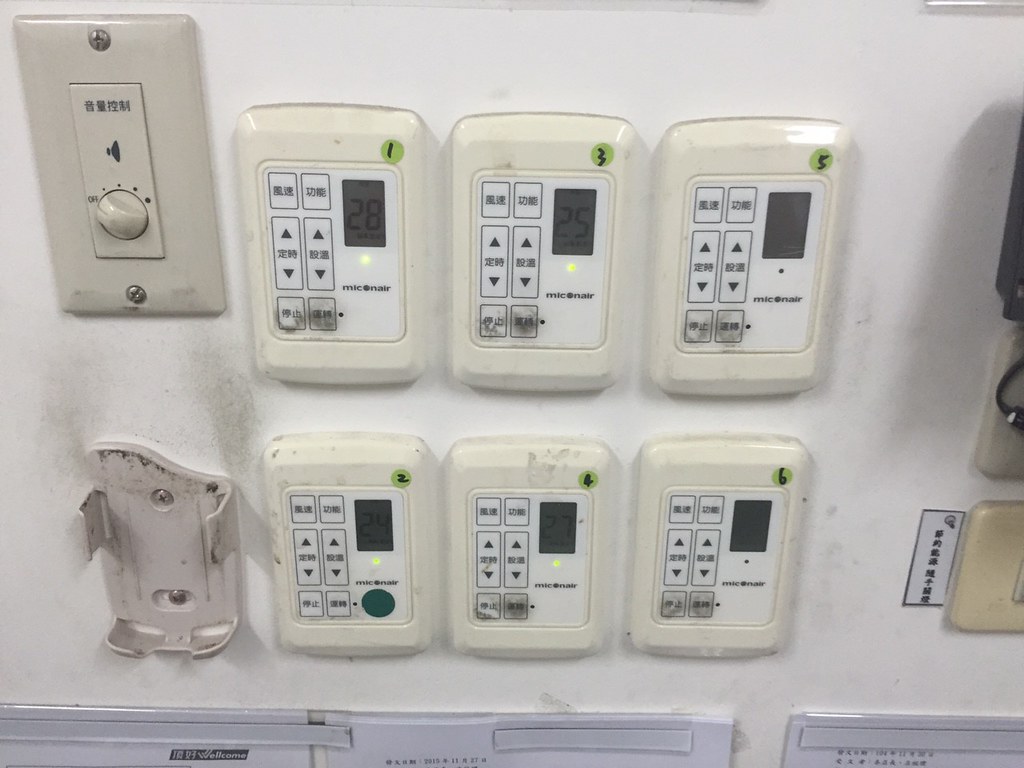The image depicts a pristine white wall adorned with a structured arrangement of various control panels. There are six controllers set into the wall, aligned in two rows of three, with each unit's face slightly protruding. The devices appear to be temperature or meter regulators. On the top row, the panels are labeled sequentially from left to right as 1, 3, and 5. The bottom row, also moving left to right, is labeled 2, 4, and 6. Each panel features a small LCD displaying black numbers, primarily showing values around '25', '26', and '28', although one unit lacks a visible display. The controllers are off-white, blending seamlessly with the wall, but their control interfaces are white with green lights indicating operational status. Touchscreen elements are present with up and down arrow buttons, alongside perforated touch-type buttons.

Additionally, a distinct gray switch plate to the right with a single round knob in the middle serves as a timer, marked with a speaker icon indicating audio functionality. Above this gray plate, there are controls with perforated touch-type buttons. There’s some writing in Japanese kanji, reinforcing its appearance as a complex control setup. A missing component is hinted by a mounting bracket on the far bottom left.